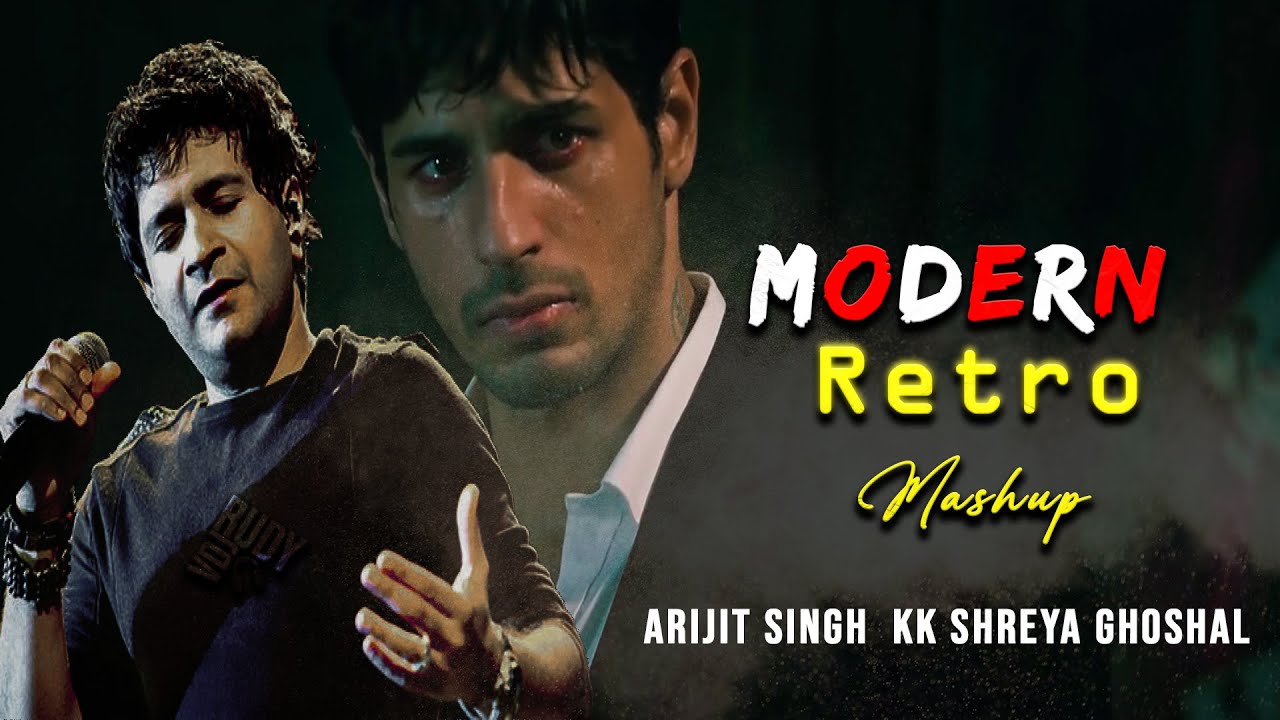The image is a horizontally oriented rectangular advertisement, possibly for a new album or concert featuring an Indian singer. The background is primarily black, fading to a cloudy gray in the middle. On the left side, there is a photograph of a man with short, curly black hair and dark skin, dressed in a black t-shirt and several bracelets. He holds a microphone in his right hand, eyes closed, with a pained expression, as if he is deeply engrossed in singing. Behind him, there's another image of what may be the same man, but this one looks skinnier and is dressed in a black blazer over a white button-down shirt with an open collar. This second figure appears to be looking off to the right, also with a distressed or emotional expression. The image includes stylized text on the right side: the word "Modern" in alternating white and red letters, "Retro" in yellow, and "Mashup" in yellow cursive. At the bottom in bold white letters, it reads "Arijit Singh" and "KK Shreya Ghoshal," likely indicating the artists' names.